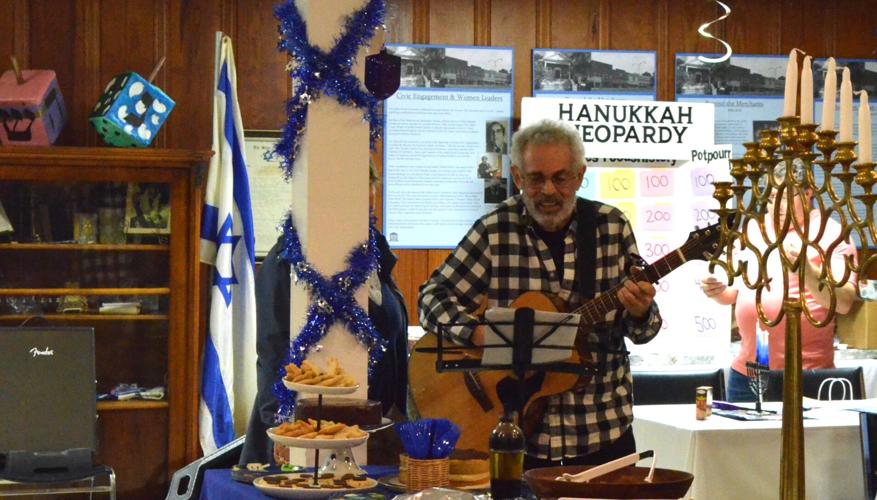The photograph captures a festive Hanukkah celebration set in a room with distinct details. Central to the scene is a man in a checkered black and white shirt, playing a brown guitar and focusing on a music stand in front of him. He's surrounded by various elements indicative of the holiday: a large menorah with partially lit candles stands behind him, and nearby, a sign reads "Hanukkah Jeopardy." To the man's left, an Israeli flag is visible, complementing the blue streamers and tinsel decorating the room. Two colorful dreidels, one pink and one blue, sit on a shelf along with various other items. There's a three-tier plate of brown cookies positioned on a white table with silverware, and a woman in a pink shirt and blue jeans stands adjacent, possibly preparing for or participating in the Hanukkah Jeopardy game. Additionally, a black chair supports a Franklin speaker, part of the cozy and intimate setup likely in someone's basement.